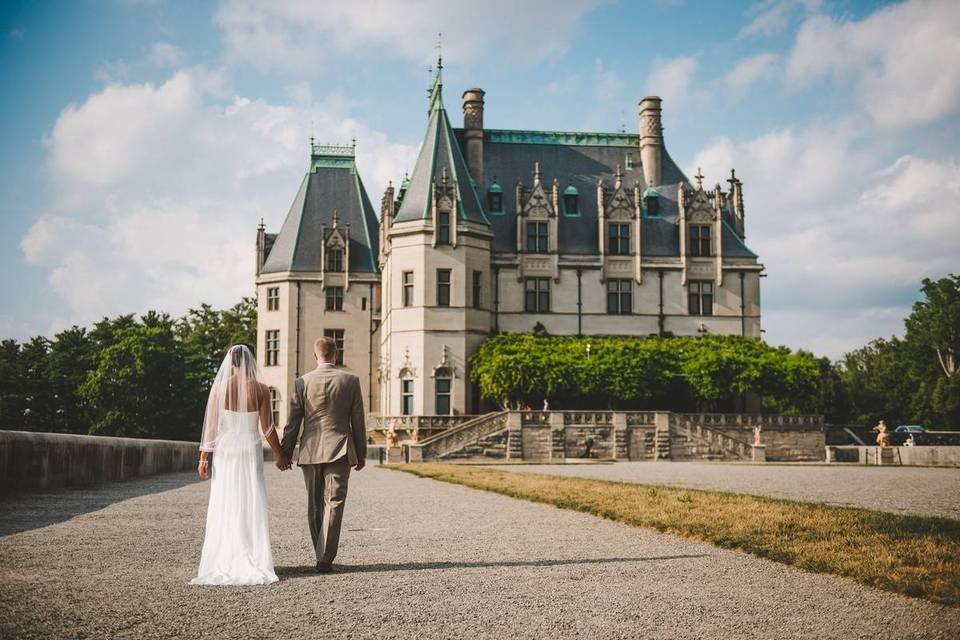A newlywed couple, a man in a grey suit and a woman in a long white wedding dress with a veil, presumably white people, are walking hand-in-hand towards a grand, older mansion that closely resembles a castle. This magnificent building, standing tall with its white exterior, features multiple windows adorned with intricate brickwork, and boasts turrets, two large chimneys, and a striking roof in varying shades of blue, with green accents at the top. The surrounding environment is a picturesque scene, marked by a beautiful, clear day with a blue sky and a few scattered clouds.

The mansion is approached via a long grey paved pathway that transitions into a gravel road, bound by a stone wall and iron fences leading up to a brick staircase with brick railings. Alongside the pathway, there's a noticeable strip of dead grass contrasted by lush green hedges and tall trees providing privacy and adding to the scenic beauty. To the right of the house stands a statue, and just behind it, partially visible in the background, is the top of an SUV. This idyllic setting is further enhanced by the greenery of trees surrounding and the well-maintained gardens that frame this enchanting abode.